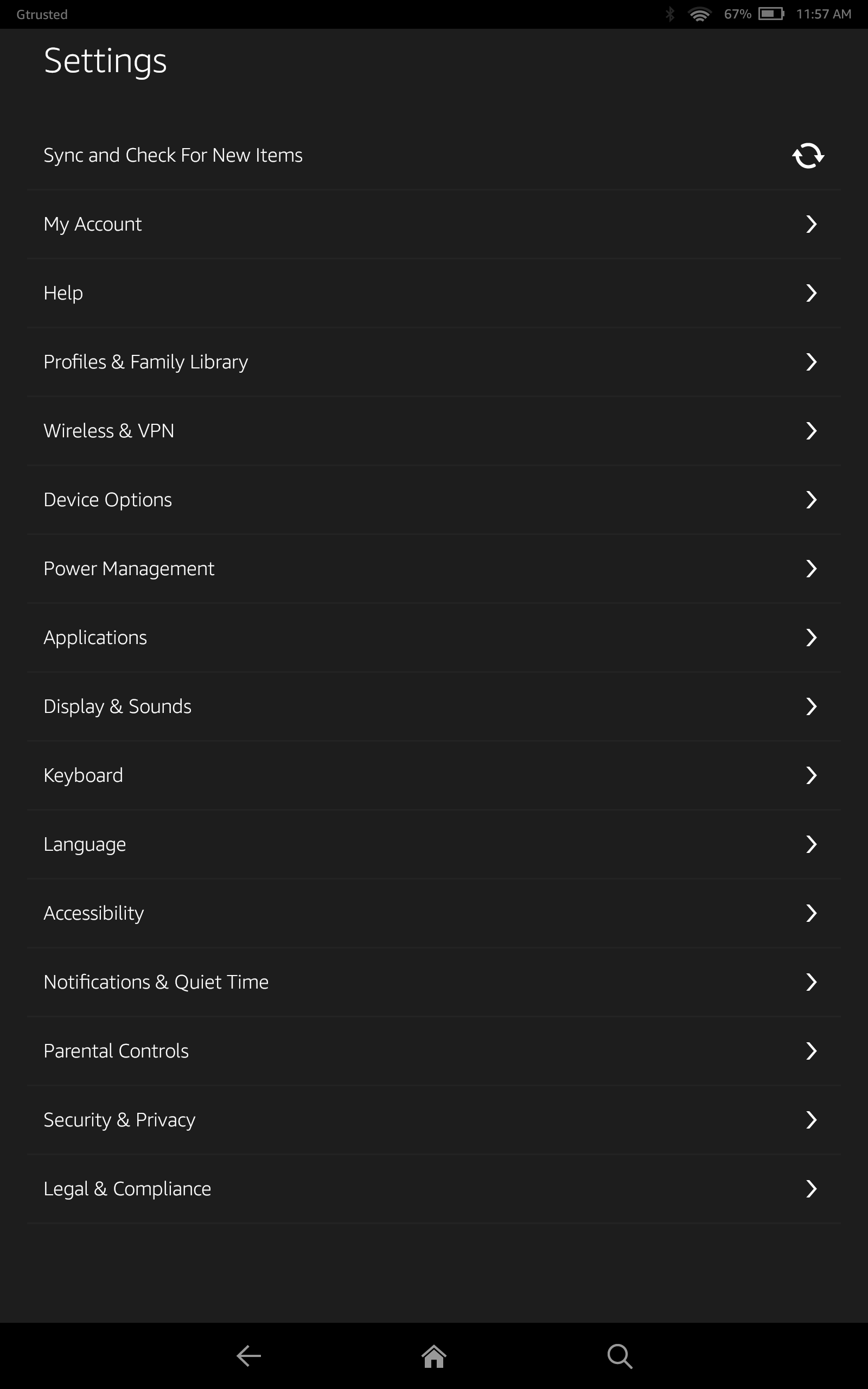The image depicts the settings menu of a smartphone screen showcasing a variety of icons and options. At the top of the screen, there are status indicators including a G-Trusted label, the Bluetooth symbol, a nearly full Wi-Fi signal, a battery icon displaying 67%, and the current time shown as 11:57 AM. The settings menu is organized into 16 rows of options. These include:

1. **G-Trusted**
2. **Bluetooth**
3. **Wi-Fi**
4. **Battery Status (67%)**
5. **Time (11:57 AM)**
6. **Settings**
7. **Text Edit Sync**
8. **Check for New Items**
9. **Refresh Button**
10. **My Account**
11. **Help**
12. **Profiles and Family Library**
13. **Wireless and VPN**
14. **Device Options**
15. **Power Management**
16. **Application**
17. **Display and Background**
18. **Keyboard and Language**
19. **Accessibility**
20. **Notifications and Quiet Time**
21. **Parental Control**
22. **Security and Privacy**
23. **Legal and Compliance**

In the background, a navigation bar features a left arrow, a home icon, and a magnifying glass, likely representing back, home, and search functions respectively. The bottom of the screen has a black strip, possibly indicating an area for additional navigation or touch inputs. The overall setting looks like a highly detailed and structured interface of a mobile device’s settings application.